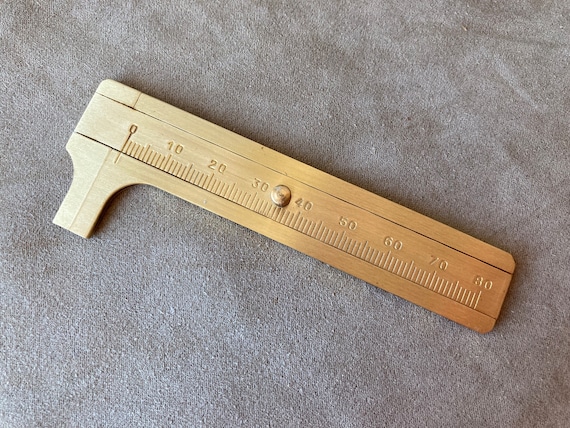The image features an antique, gold-colored metal ruler placed diagonally on a textured, light sandy brown suede background. The ruler, which appears shiny and somewhat reflective, is marked with measurements from zero to 80, with increments of ten prominently displayed, suggesting a metric system. The ruler also includes intricate detailing such as a small, curved notch resembling a high heel on the left bottom side. Towards the middle of the ruler, there is a circular, gold pin or knob, which seems to facilitate movement along a channel in the ruler, allowing precise adjustments. The suede background, with its random marks and texture, adds a subtle but rich context to the overall aesthetic of the antique measurement tool.